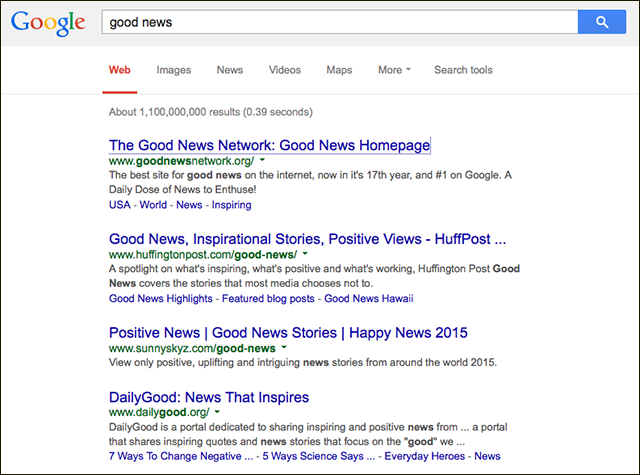The image depicts a Google search results page with a clear blue-themed interface and a magnifying glass icon. The search term "good news" is highlighted in red text. The search yields approximately 1,100,000,000 results in 0.39 seconds. Displayed prominently is the official homepage of 'Good News', available at www.goodnews.wordpress.org, celebrating its 17th year as the top source for positive stories, ranked number one on Google.

Highlighted results include various sources for uplifting news, such as Huffington Post’s Good News section, which emphasizes inspiring stories, positive developments, and health news. There is also a mention of Sunny Skies, which focuses on heartwarming stories from around the globe, and Daily Good News, dedicated to sharing daily positive news updates. Both sites are committed to highlighting everyday heroes and scientifically-backed ways to improve well-being.

The image is peppered with various content types, arranged in different text styles and formats, to emphasize the diverse range of good news sources and stories available online.